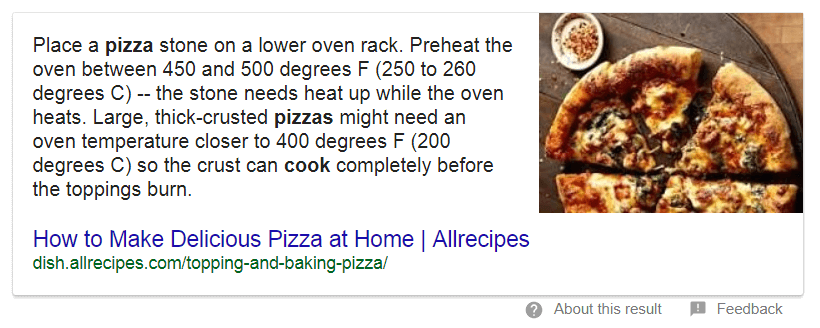The screenshot showcases a preview of a website with a detailed guide on making pizza. The horizontal image features a thin gray border, framing two distinct sections. 

On the right-hand side, there's a close-up of a freshly baked pizza resting on a brown serving platter, placed atop a wooden tabletop. The pizza, sliced into six pieces, boasts a thick, puffy brown crust. The toppings include melted yellow cheese, bits of mushrooms, and a layer of rich sauce, suggesting a savory and appetizing meal. Adjacent to the pizza, on the top left, there's a small white dish containing a seasoning that appears to be garlic or some other brown powder, adding to the rustic and flavorful presentation.

The left-hand side of the image transitions into a white background featuring black text. The text provides a step-by-step guide for baking pizza: "Place a pizza stone on a lower oven rack. Preheat the oven between 450 and 500 degrees Fahrenheit (250 to 260 degrees Celsius). The stone needs to heat up while the oven heats. Large thick-crusted pizzas might need an oven temperature closer to 400 degrees Fahrenheit (200 degrees Celsius), so the crust can cook completely before the toppings burn." Below this informative text, a blue hyperlink is presented: "How to make delicious pizza at home from Allrecipes." The URL provided is dish.allrecipes.com/topping-and-baking-pizza.